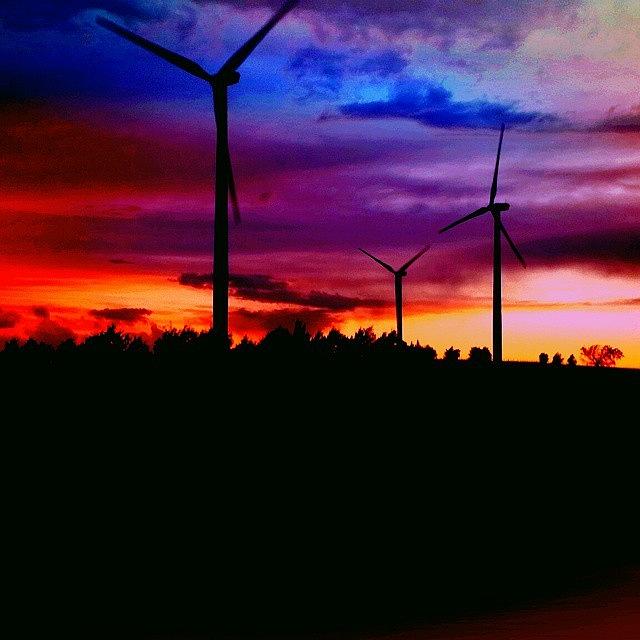This vivid color photograph, presented in a square format, captures a serene yet dramatic sunset scene at a modern wind farm. The sky, painted with an array of vivid hues including fiery oranges, reds, purples, and blues, hints at the moment just after the sun has dipped below the horizon. Scattered clouds reflect this vivid light, creating a breathtaking and fiery backdrop. Dominating the image are three wind turbines, standing in silhouette against the vibrant sky, their blades slicing through the dynamic colors. In the foreground, on the left, a large wind turbine stretches upward, its blades extending near the top left of the image, with one blade tantalizingly cut off. To the right, two smaller turbines are visible, receding in size due to their distance, with the medium one on the right and the shortest near the center. The lower half of the photograph reveals a landscape in complete shadow, featuring a line of indistinct trees or bushes that form a dark horizon. The photograph, embracing a style of realistic representationalism, beautifully captures the juxtaposition of human ingenuity and natural splendor, framed in a moment of tranquil dusk.